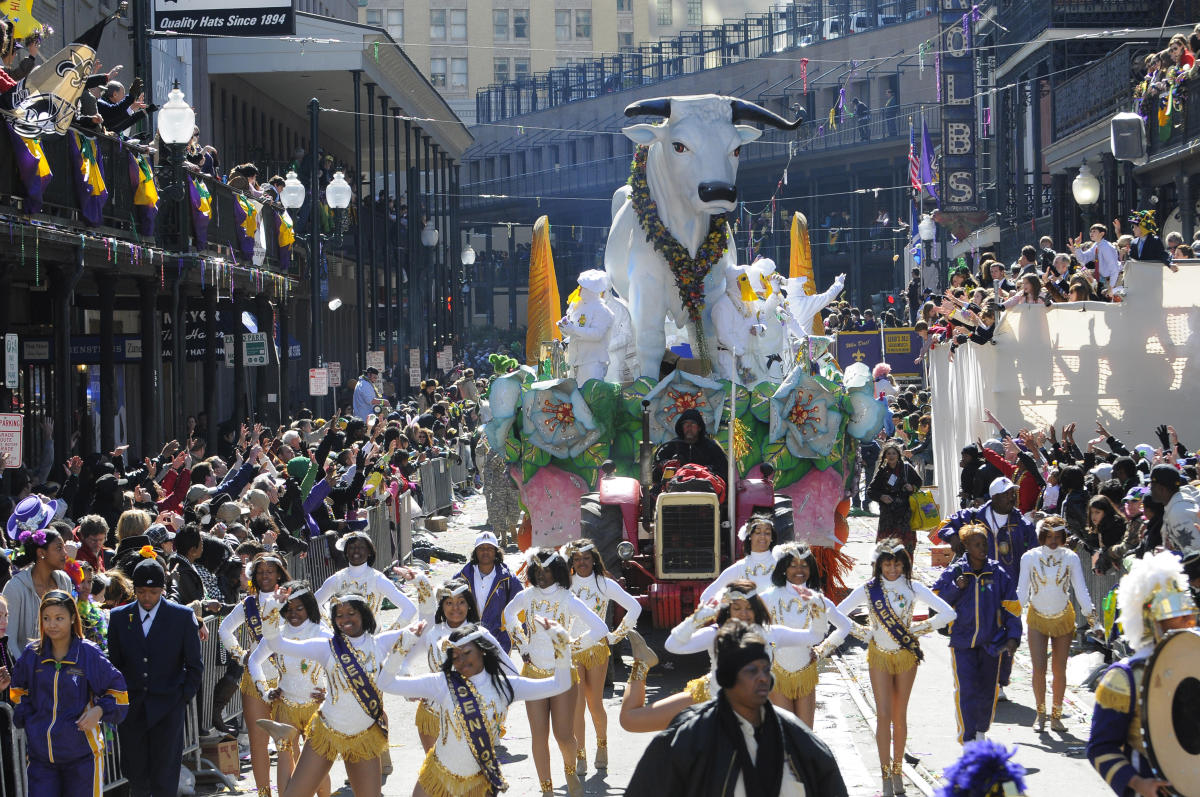The photograph captures a vibrant and bustling parade scene. In the foreground, African American women and others dressed in white leotards with gold skirts and some in blue tracksuits with gold stripes dance energetically. A red tractor, adorned with a giant figure of a white bull featuring black horns, a black nose, and a multicolored floral wreath made of paper mache flowers in yellow, pink, red, and orange with green leaves, dominates the center of the image. Surrounding the float, numerous spectators line both sides of the street; on the left, people wave from a black balcony while on the right, silhouettes of individuals are visible through thin white walls covering bleachers. Toward the back, some revelers stand atop another banister. The street is flanked by various businesses, enhancing the urban carnival atmosphere. Celebratory energy permeates the scene, with others visibly cheering, waving, and capturing moments on their phones amidst the lively crowd.